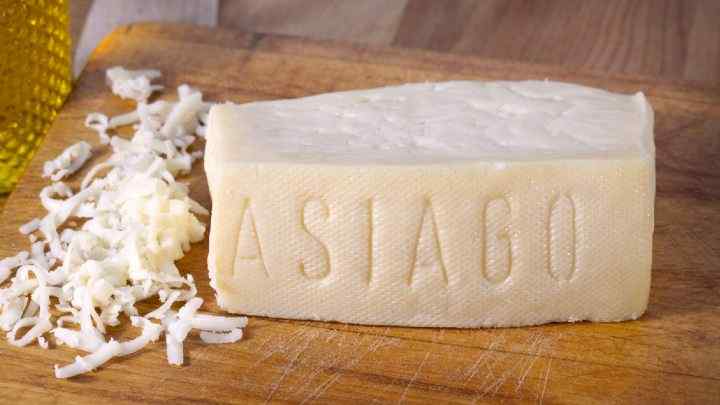In the image, a large rectangular block of Asiago cheese sits prominently on a brown, heavily scratched cutting board. The middle of the block features the word "ASIAGO" chiseled in all capital letters. To the left of the block, there are scattered light yellow to almost white shreds of the cheese, indicating that part of the block has been shredded. The cutting board, which may be on a wooden table, has noticeable darker brown lines and serves as the main background. In the upper left-hand corner, a yellowish-gold object, possibly a wicker basket or container, is partially visible, contributing to the homey setting. The top of the image shows a blurred area that could be additional countertop space or another cutting board in the background.